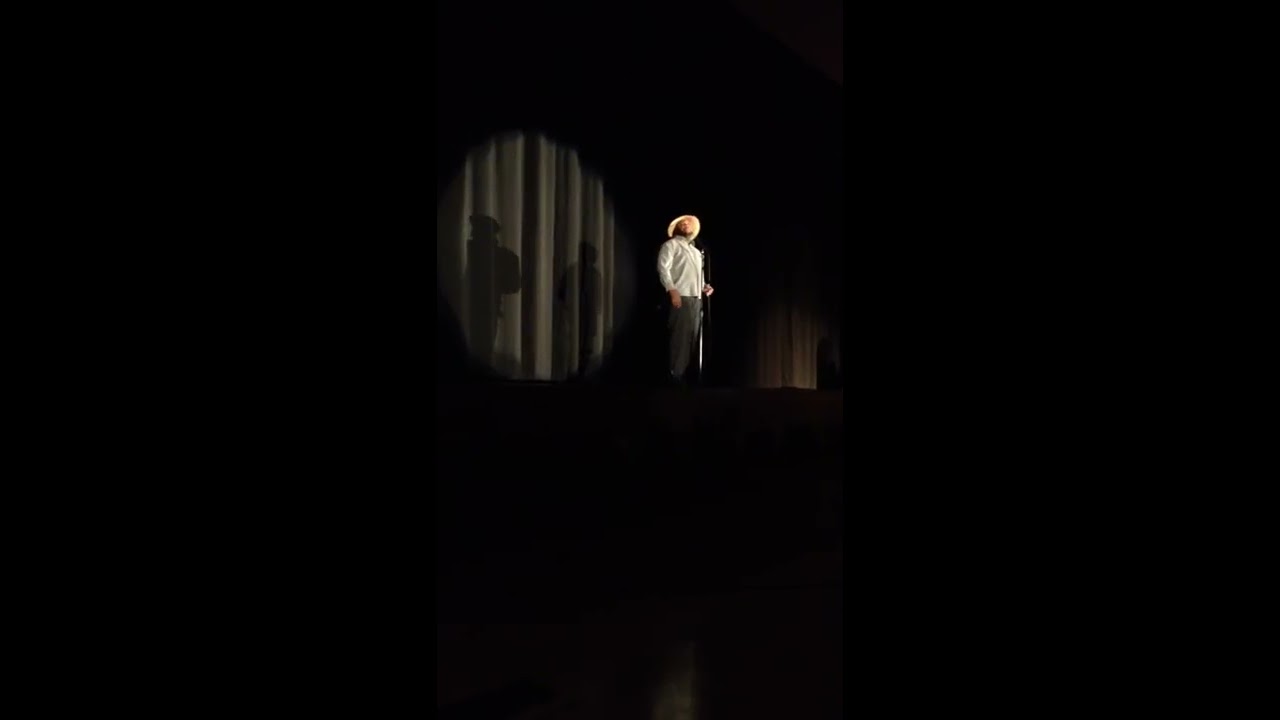In the image, a lone African-American performer stands on an elevated stage, about eight feet above the unseen audience, bathed in a bright spotlight that sharply contrasts with the dark background. He is adorned in a wide-brimmed straw hat, a light-colored long-sleeve business shirt, and blue Levi's denim jeans. A microphone on a stand is positioned in front of him, suggesting he might be a stand-up comedian. Behind him, an olive-green curtain partially illuminated by an amber side light hints at instructions for his exit. The stage's faint background features his shadow contrasting against the dark, otherwise indistinguishable surroundings. In the distance, only a single audience member's shadow is faintly visible among the rows.